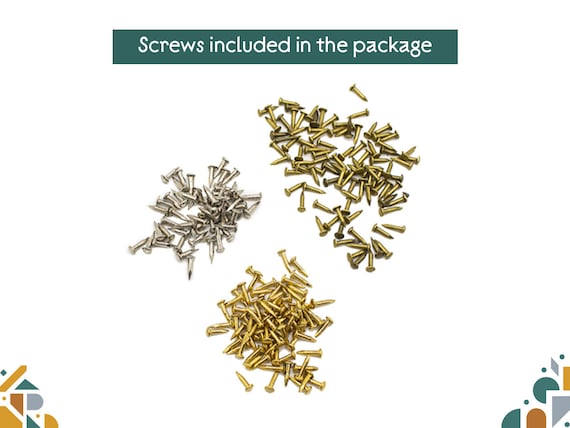The image features a clean white background with decorative geometric shapes in the bottom right and top left corners. These shapes include half-circles, circles, triangles, and rectangles, rendered in a palette of green, tan, brown, and gray. A green bar with white text at the top of the image reads "Screws included in package." Below this text, scattered across what appears to be a white tabletop, are multiple sets of tiny screws. These screws are differentiated by their colors and materials; there are brass screws, silver screws, and bright brass screws all neatly arranged on the white surface.